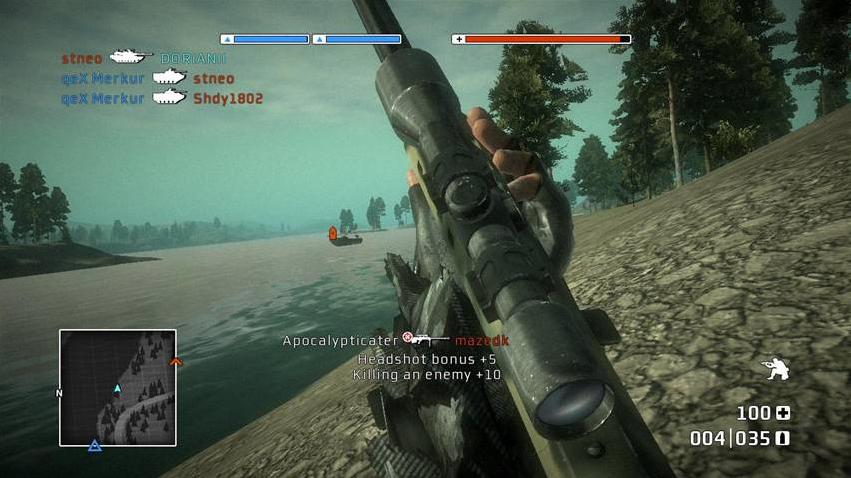This image is a detailed screenshot from a first-person shooter video game. Dominating the foreground, a camouflage-colored rifle is firmly gripped by a visible right hand, suggesting the player’s perspective. The rifle is centered prominently at the bottom of the frame. The background reveals a desolate, desert-like terrain characterized by a sandy, grayish-brown hue. The horizon is sparsely populated with distant trees, giving the scene a barren and isolated atmosphere. The sky above is hazy, tinted with a subtle aqua blue. To the upper right corner, a cluster of pine trees stands out against the skyline. The lower right-hand corner showcases a patch of rugged, rocky terrain. Overlaying the scene, text elements are visible, including the partial word "apocalypticator," and game notifications such as "killing an enemy" and "headshot bonus," indicating recent in-game achievements.